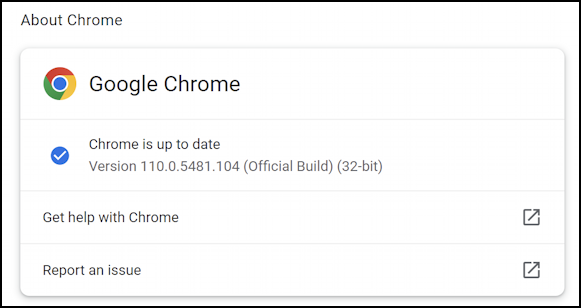The image is a screenshot of a Google Chrome update notification interface. The rectangular image features a black border at the top left corner within a gray background area. The primary section has a shadowy light gray border and rounded corners. At the top left of this section, the Chrome logo is prominently displayed—a circle with an outer border segmented into three colors: red at the top left, yellow on the right, and green at the bottom left. The logo also includes a white circular outline with an inner filled blue circle.

To the right of the Chrome logo, "Google Chrome" is written in dark gray text. A faint horizontal line serves as a divider below this heading. Underneath and towards the left, there's a dark blue circle with a white checkmark, indicating the current selection. To the right, in black text, it reads "Chrome is up to date," with the version number "Version 110.0.5481.104 (Official Build) (32-bit)" written in gray below it. 

Another faint gray divider separates this section from the next. Below it, in black text, it reads "Get help with Chrome," accompanied by a share icon—a square with an upward-pointing arrow—towards the right. Following another faint gray divider, the text "Report an issue" appears in black, also accompanied by a share icon to its right. 

The entire layout has a subtle shadow effect around its borders, providing a slight depth. The footer at the bottom of the image features a light gray background, distinct from the otherwise white background of the main interface.